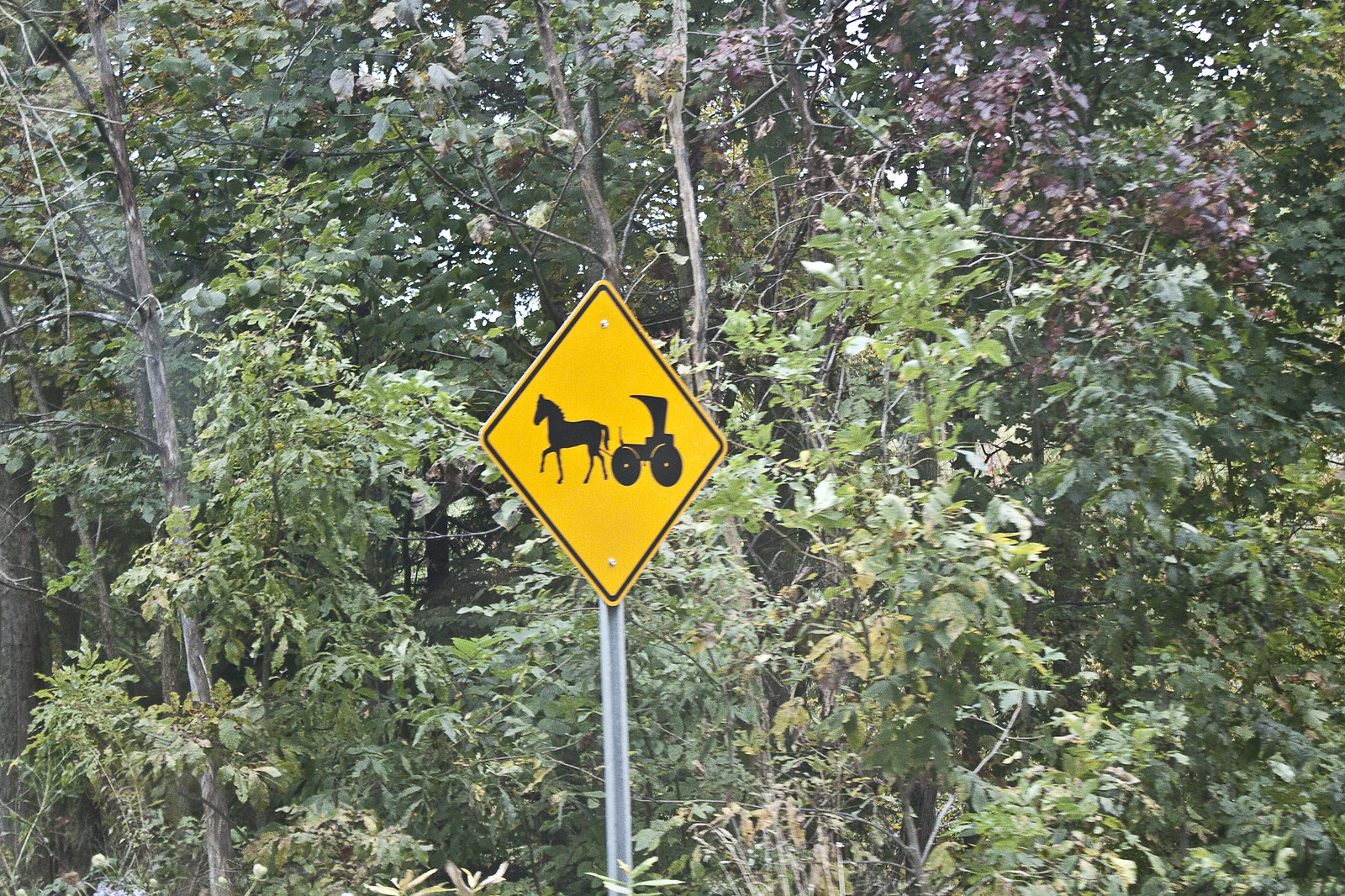The photograph features a yellow, diamond-shaped traffic sign prominently positioned at the center. The sign is outlined with a narrow black band and is mounted on a long, grey pole. Within the sign, a black outline illustration depicts a horse pulling a carriage, reminiscent of those used by the Amish. The image is framed by a forested area with tall trees adorned in primarily green leaves, though some leaves exhibit shades of yellow and purple. Sunlight filters through the dense foliage, casting whitish-grey points of light. The viewpoint suggests the photo was taken from a slightly upward angle, emphasizing the height of the trees. The scene is well-lit, indicating it was taken during daytime, with hints of bluish sky visible through the leafy canopy. The ground beneath the sign is not visible in the image.